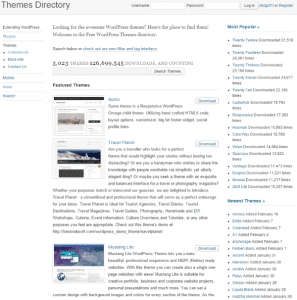A screenshot of a computer screen is displayed, featuring a highly detailed interface dense with information. At the very top, a light gray navigation bar is prominently labeled "Themes Directory," accompanied by a couple of white search fields on its right side. Below this, on the left, there appears to be a table of contents with clickable blue text. The central area of the screen represents the main content section, overflowing with textual information. Within this section, there are two images located on the left; the lower image is partially cut off, while the upper one is quite small, suggestive of a newspaper layout with text wrapped around the images. On the right side of the screen lies a third column filled with blue hyperlinks and bullet points extending down the page, indicative of various navigational links. The bottom image in the content area also features a touch of purple in its top-left corner. Overall, the color scheme of the screen is predominantly black and white, with occasional accents of blue text, contributing to an organized yet densely packed presentation of information across detailed paragraphs.